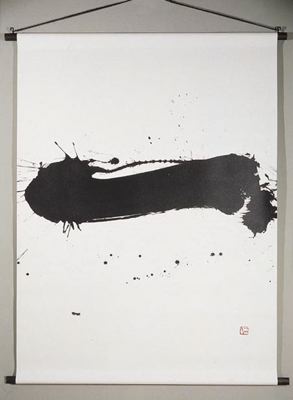This image captures a highly abstract piece of art displayed on a white scroll. The photograph's background is gray, and the scroll itself is suspended from a hook or nail, likely by a black string, giving it an almost suspended, floating appearance. The scroll unfurls vertically, anchored by two black poles at its ends.

On the scroll, a dramatic, disorganized splash of black ink dominates the composition, with the primary streak stretching mostly horizontally across the paper. This central, chaotic brushstroke is accompanied by numerous smaller black dots scattered around it, creating a sense of movement and energy. The ink appears thick in certain areas, causing it to splatter and run, adding a dynamic texture to the artwork.

In the bottom right corner of the scroll, a distinct red square shape can be seen, possibly acting as a signature or an artistic accent, contrasting starkly with the monochrome black and white of the rest of the piece. The artwork is lit from the front, highlighting the ink's texture and the scroll's creamy white surface. Overall, the image presents a compelling mix of controlled structure and wild expressiveness.